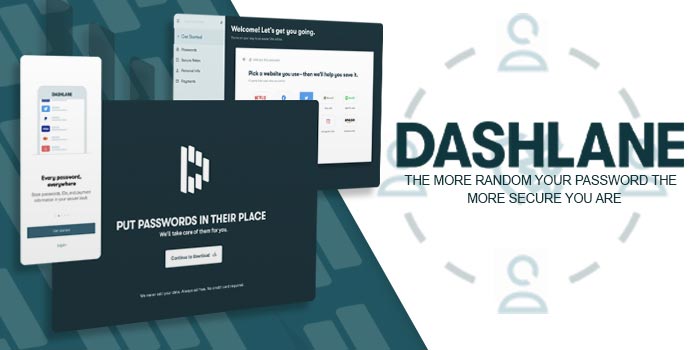This is an advertisement for Dashlane, an app designed to enhance password security. The image is divided diagonally into two sections: the left side features a teal background with a pattern of lighter teal blocks, while the right side has a clean white background. On the right, the Dashlane logo is prominently displayed with the tagline, "The more random your password, the more secure you are." Overlaying the background is a dashed circle with iconography representing people, and a subtle, partially obscured lock symbol indicative of security.

On the left side, a series of tilted, rounded-rectangle screen captures illustrate various pages and features of the app. These mobile and website screenshots are digitally rendered to give a dynamic, angled perspective, creating the illusion of depth and motion. The overall design balances textual information with visual elements, conveying a message of advanced digital security through a modern and visually engaging layout.